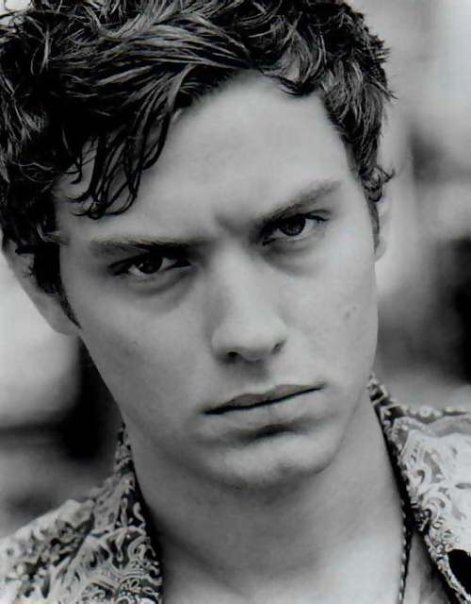The image is a high-contrast black and white photo of a younger man, possibly actor Bill Skarsgård, staring intensely at the camera. His expression is serious, with a noticeable frown and crinkled forehead which highlights lines between his eyebrows. The man has short dark hair that is longer on the top, styled in a slightly messy manner with a mousse-like texture, and long sideburns. He is clean-shaven with a chiseled face, and a small mark is visible on one of his cheeks. He is wearing a patterned shirt, possibly a Hawaiian or paisley print, with a collar. A chain necklace peeks out from the neckline of his shirt, though it is partially cut off by the framing of the photo. The background is a blurred-out gray gradient, providing no discernible details, and the depth of field focuses sharply on the man's face and shoulders, which are the only parts of his body visible in the image. The overall clarity and brightness of the photo make the subject and his intense gaze stand out vividly.